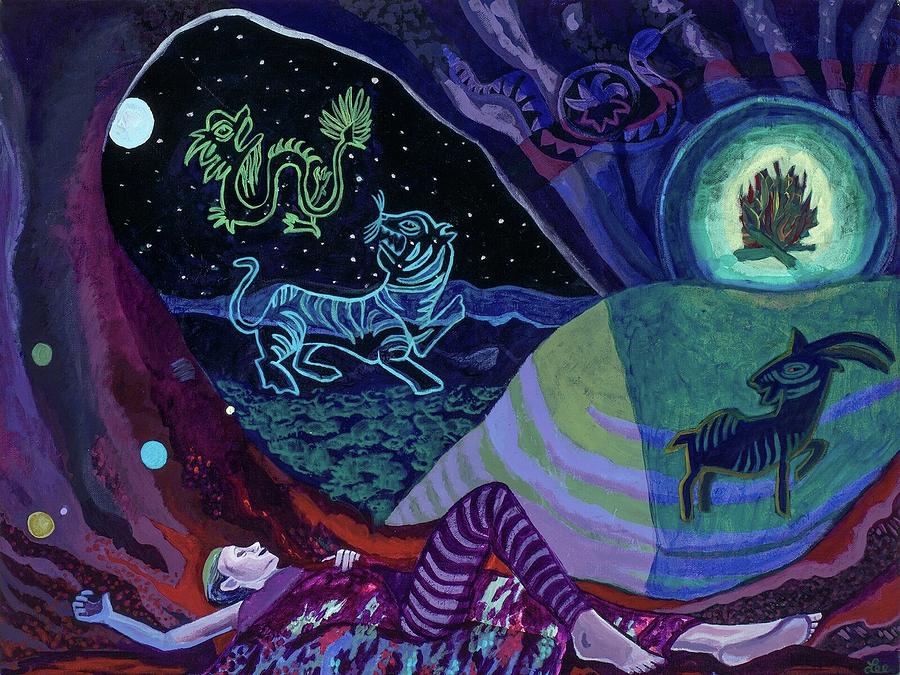This vivid cartoonish illustration appears to be drawn with fluorescent or neon-colored chalk on a black surface, giving it an ethereal glow as if illuminated by a black light. The scene is set inside a cave with walls shaded in dark and light purples, accented with touches of red. The cave interior features various mystical elements: to the right, there are primitive drawings including a black deer, a campfire with two pieces of wood, and what seems to be a goat. 

Laying on the ground inside the cave is a figure, possibly a woman, dressed in light and dark purple striped pajama pants. She is barefoot, her right arm resting beside her head, and a blanket or shawl draped over her as she lays flat on her back with one knee bent.

Outside the cave, the night is captured in a strikingly detailed manner. The sky is a deep black, dotted with stars, and illuminated by a prominent moon positioned to the left. Against this celestial backdrop, a series of vibrant creatures come to life. A green dragon hovers in the upper left-hand corner, below which a blue tiger prowls. In the upper right corner, a blue snake-like creature winds its way across the scene, adorned with a round marking on its back. This fantastical depiction combines elements of reality and imagination, creating an enchanting visual narrative.